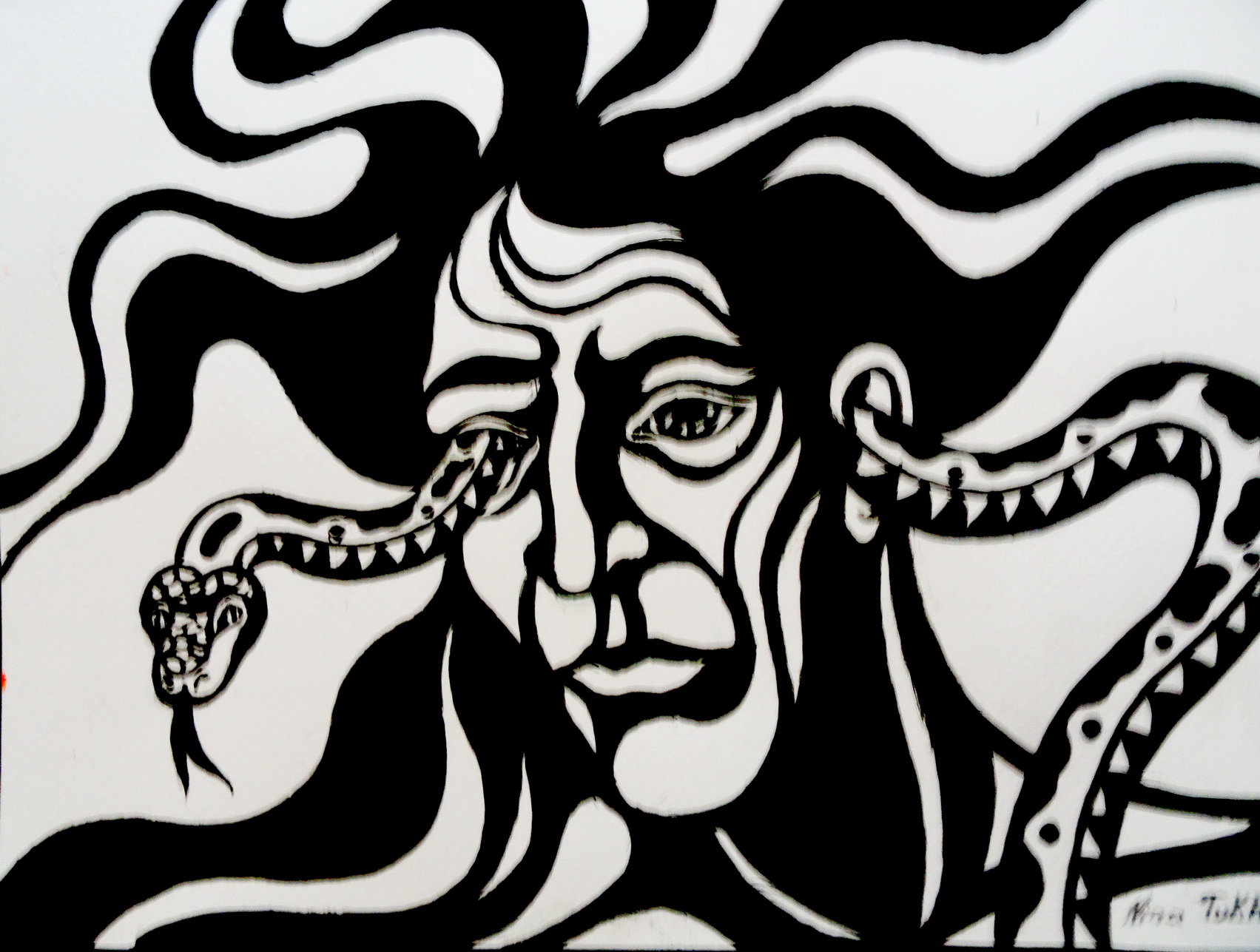This black and white graphic art piece depicts a person with wavy, wild hair that resembles the serpentine locks of Medusa. The striking image features a snake with intricate patterns of triangles, circles, and blotches, weaving through the person's left ear and emerging from their right eye. The snake is hissing, its black, forked tongue fully extended. The face of the figure is detailed, showing both eyes—one intensely penetrated by the snake—along with a defined nose, mouth, and lips. The figure appears expressionless, gazing distantly, and the wavy lines of the hair continue to swirl around parts of the face, enhancing the eerie and surreal quality of the artwork. Additionally, the artist's signature is located in the bottom right corner, though it is indistinct.